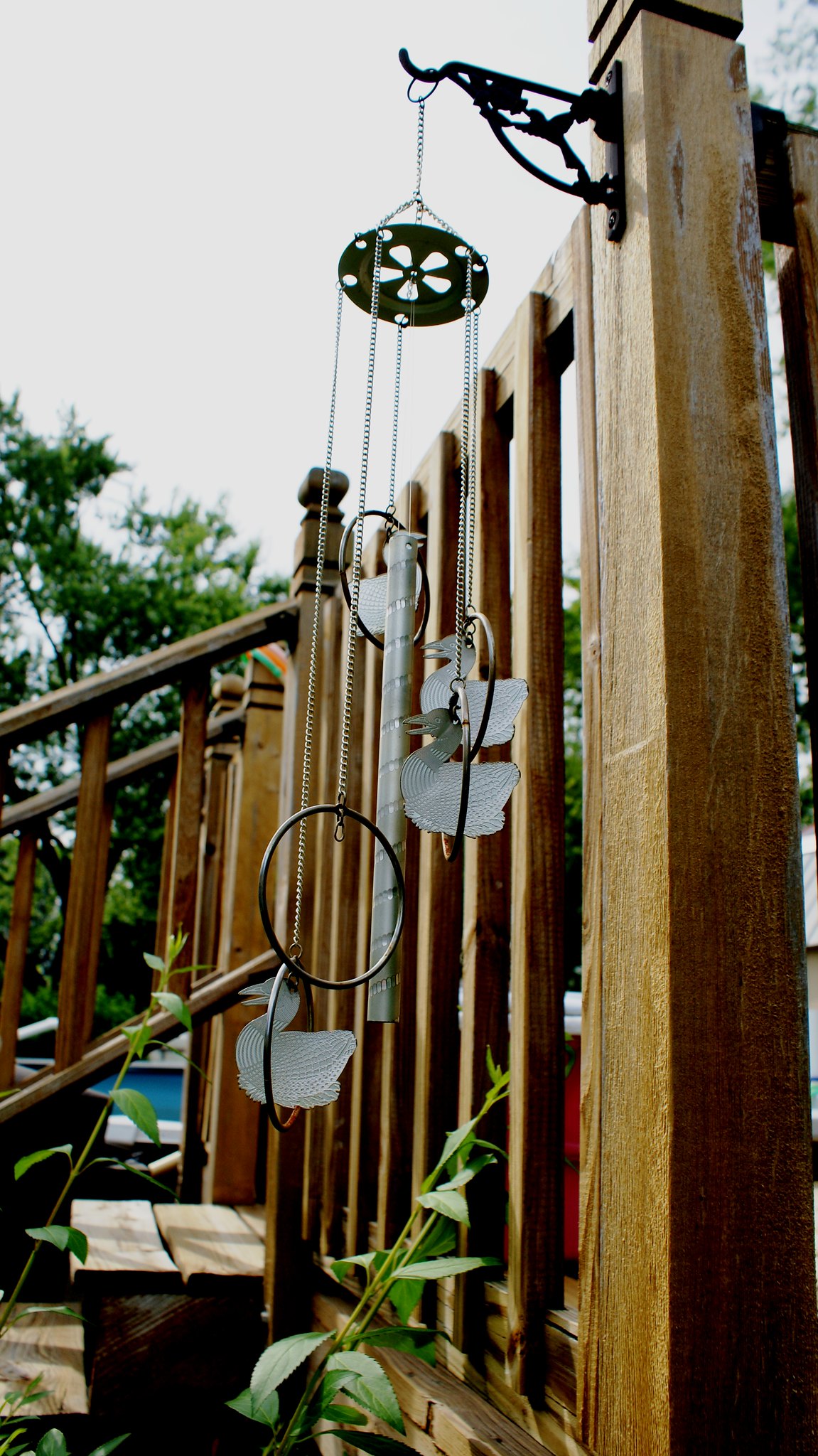This vibrant color photograph captures an artistically designed wind chime hanging from the corner of a wooden deck. The vertical, rectangular image highlights a post in the foreground on the right-hand side, where the chimes are attached. The chimes are intricate, featuring a round metal top adorned with a daisy cut-out pattern, from which multiple chains descend. These chains support several large brass-colored circles and cut-out figures of ducks, likely made of cut aluminum, designed to create soothing sounds when swayed by the wind. 

The deck, constructed of red-colored wood, possibly redwood, features vertical slats and steps that lead downwards to the left. Mounted atop the post is a black wrought iron hanger, embellished with a bird figure, possibly a hummingbird. Below the wind chimes, a small green plant is thriving around the base of the post. 

The background reveals a wooden fence extending across the frame, a small tree, and two steps with a railing. The sky above is overcast and gray, enhancing the tranquility of the scene. Additional elements include a red container with a white lid positioned on the decking, a blue object that might be a vehicle, and a green bin, providing a glimpse into the everyday life surrounding this serene setting.